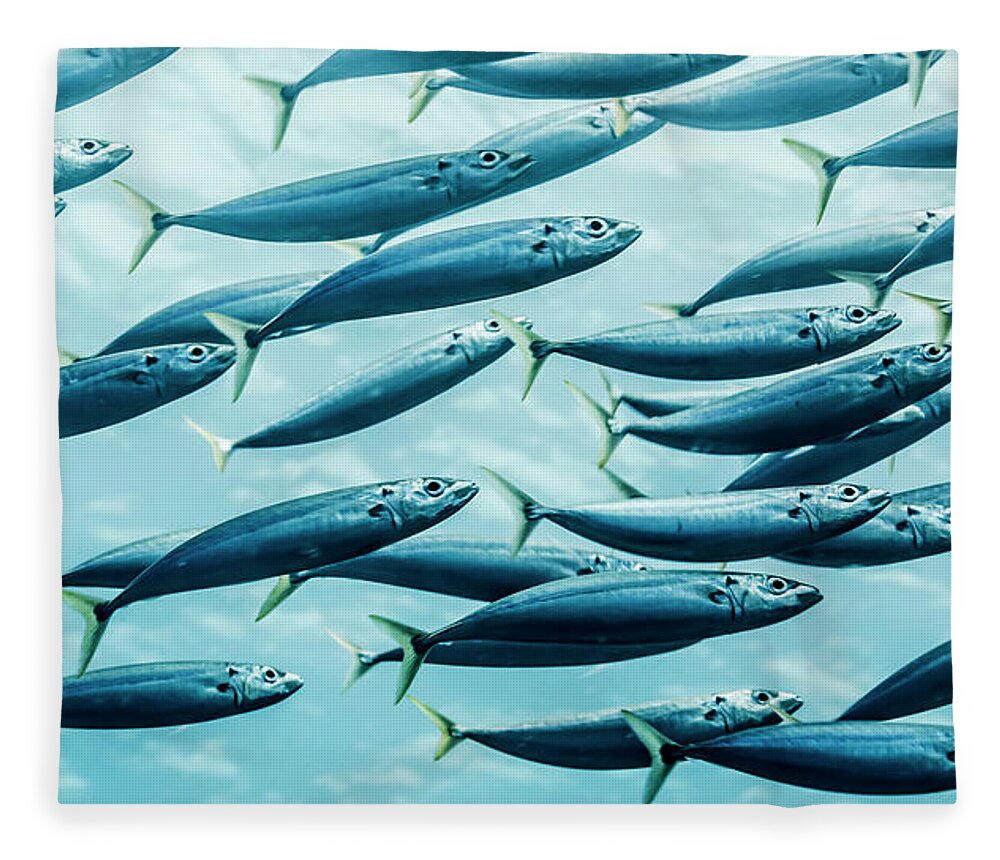The image depicts a close-up view of numerous small, slender, schooling fish swimming together underwater, all uniformly oriented from left to right. They bear a bluish-silver hue with a greenish tint on their tails, and their bodies are long and thin, reminiscent of sardines or anchovies. The fish have notably large, bright eyes with black centers, positioned near their small, almost indistinguishable gills. They lack dorsal fins, with their only visible fin being the one on their tail. The background consists of a gradient of light blue tones, becoming darker towards the bottom, creating a watery effect that suggests daylight reflection from above. The overall color scheme of the image blends the fish seamlessly with the background, enhancing their aquatic environment. The picture captures approximately 20 to 25 fish, some fully visible while others are partially cut off, making it appear dense and vibrant with marine life.